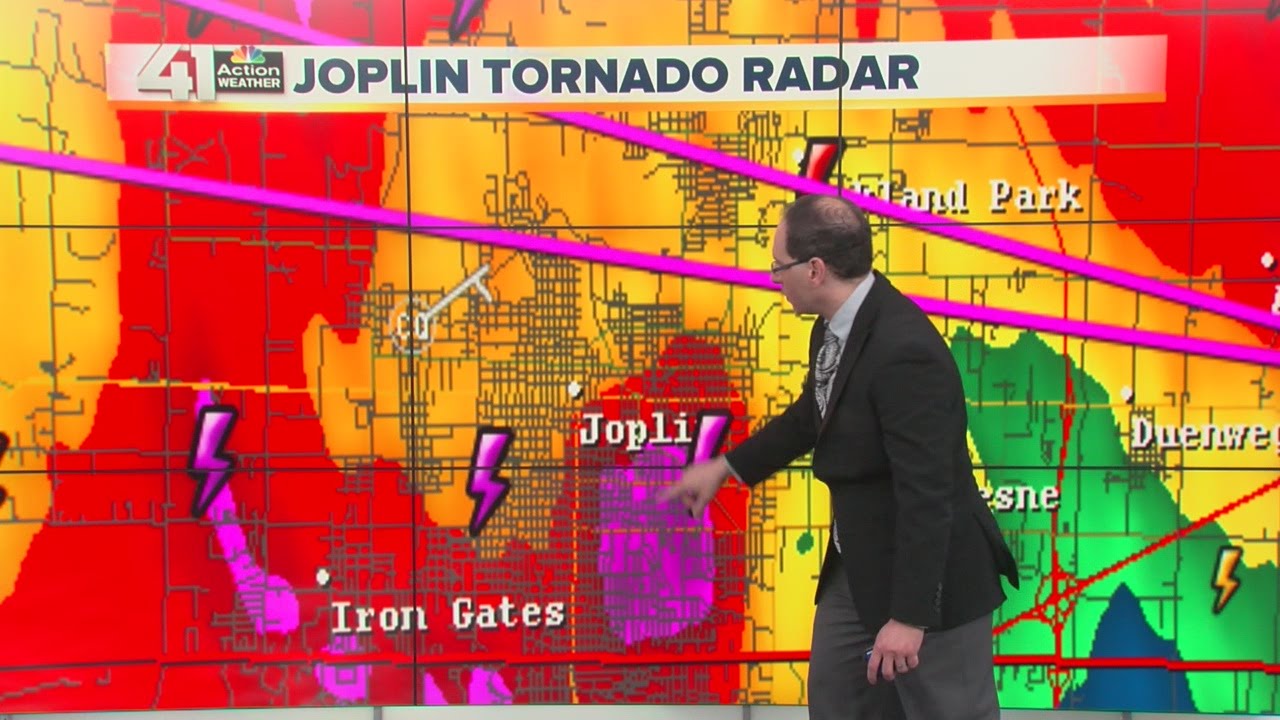The image is a rectangular horizontal scene from a weather report featuring a vividly colored map on the wall. At the top of the image, a white banner reads "Action Weather, Joplin Tornado Radar," accompanied by an illegible logo to its left. The focal point is a man with short brown hair and a bald spot, wearing glasses, a dark suit coat, a light blue shirt, a tie, and gray pants. He is pointing to a predominantly purple area on the map labeled "Joplin," which is surrounded by a significant red region indicating severe weather. The detailed map also highlights lightning symbols and a grid layout of city streets above Joplin. Below Joplin, an area labeled "Iron Gates" can be seen, though other nearby labels are obscured by the man's position.